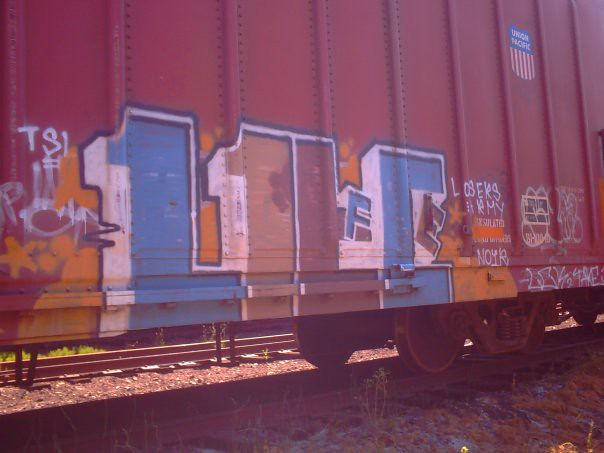This detailed, horizontal rectangular photograph showcases a partial view of a burgundy train boxcar adorned with graffiti and the iconic Union Pacific emblem—a blue shield with red and white stripes and "Union Pacific" written in white. The image highlights the boxcar's undercarriage, where four wheels rest on the train tracks, framed by scattered pebbles, brown dirt, and a hint of grass in the background. Trailing behind are additional train tracks.

Prominent graffiti on the side of the boxcar features large, 3D block letters "L1LC" spanning vertical rectangular sections, with the Ls in blue and reddish-brown, the 1 in a brownish hue, and the C in blue. Among the graffiti, the white and yellow paint stands out, particularly a small yellow star and the phrase "TSI =" in white. Another striking piece reads "Losers are my noir" in white paint. The detailed artwork and textures of this vibrant scene capture the blend of industrial utility and street art.